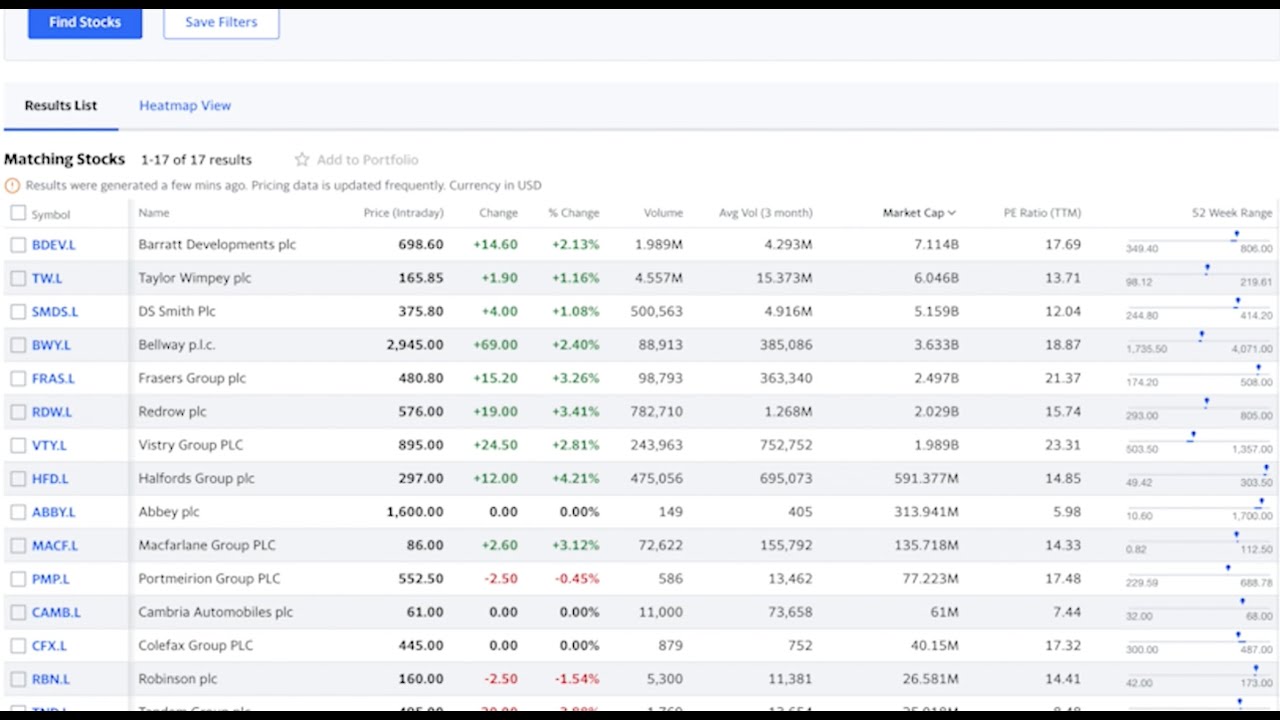Here is a cleaned-up and detailed caption:

---

This screenshot is taken from a financial website, capturing a detailed view of a stock listing page. The image is bordered by black lines at the top and bottom. Just below the top black line, there's a distinct light blue rectangle. In the upper left corner of this rectangle, a blue button with the white text "Find Stocks" is prominently visible. Adjacent to it, on the right, a white button with blue text reads "Save Filters." Below these buttons lies a horizontal white line, further followed by another blue rectangle that dominates the content area.

In the upper left corner of this second blue rectangle, black text declares "Results List," indicating the selected tab. Directly beneath this, a blue horizontal line separates it from the list view options. To the right, blue text displays "Heat View Map," offering an alternative visual representation of the data.

Beneath this setup, the list commences, headlined by a section labeled "Matching Stocks 1 through 17 of 17 results." Alongside this header is a small, five-pointed star icon accompanied by the option "Add to Portfolio." Underneath this header, gray font provides additional context: "Results are Generated a Few Minutes Ago. Pricing Data is Updated Frequently, Currency: USD." 

Continuing further down, a vertical list features in the left column, marked by stock symbols in blue font including BDEVL, TWL, SMDSL, BWYL, FARSL, RWEL, VTYL, HFTL, and ABBYL.

---